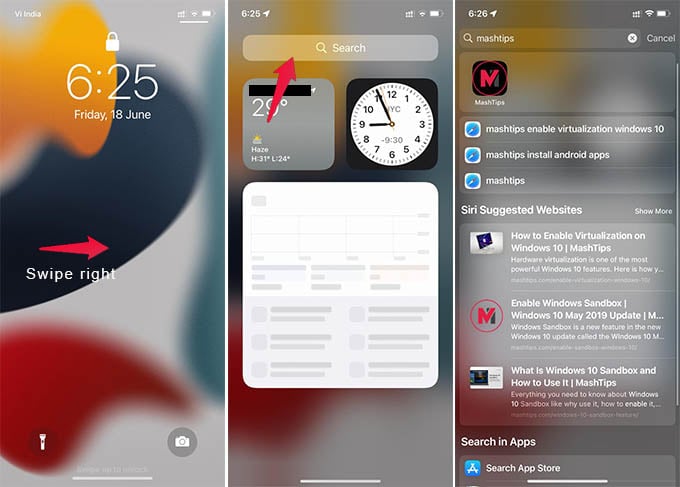This image is a three-panel display of someone's phone screen. The carrier listed at the top is WI India. The left panel shows the lock screen, indicating that it is 6:25 on Friday, June 18th, with approximately 80% battery remaining. The lock screen features an abstract wallpaper with colorful shapes on a black background, including a partial yellow circle and a red hat-like shape. A red arrow and text prompt "Swipe right" are also present.

The middle panel displays the home screen, featuring a search bar at the top, which is light gray against a darker gray background with abstract shapes. Below the search bar are various widgets. The first widget is the Weather app, showing a temperature of 29°C and hazy conditions, with the city name obscured. Another widget displays the time as 8:55. There is also a large, light gray, off-white rectangle widget, the contents of which are not visible.

The right panel displays the results for a search query "mash tips." The main result is the app icon for MashTips, which is black and red. Below it are search suggestions related to MashTips, including "enable virtualization Windows 10," "install Android apps," and more. Siri's suggested websites for enabling virtualization on MashTips are listed below these suggestions. At the bottom of the screen, there is an option to "search App Store" with the App Store icon.